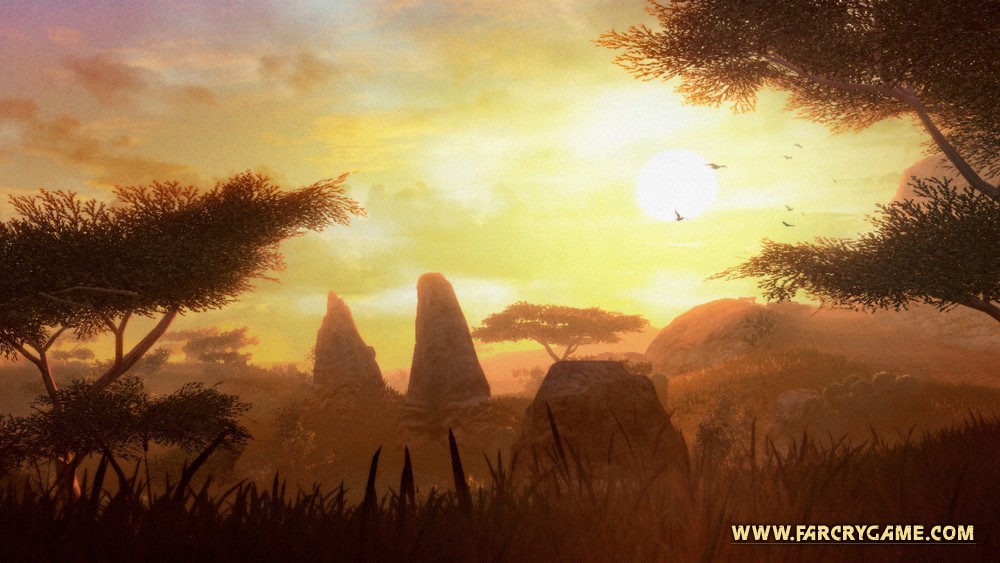This image is a screenshot from the video game Far Cry, as noted by the text "www.farcrygame.com" in the bottom right corner. The scene captures an African plains landscape under a predominantly yellow sky, suggesting either a sunrise or sunset, with hints of gold and a touch of red in the upper left corner. The foreground is characterized by dark brown and light brown earthy tones, with clay-colored rocks blending into the terrain. The mid-ground features various trees, some large with expansive branches covered in leaves, acting as a natural frame for two significant rock formations in the distance. Birds can be seen flying across the sky, adding life to the scene. The overall image gives a muted, serene atmosphere, with the sun casting its reflection, amplifying the sense of calm and natural beauty in this expansive jungle-like setting.